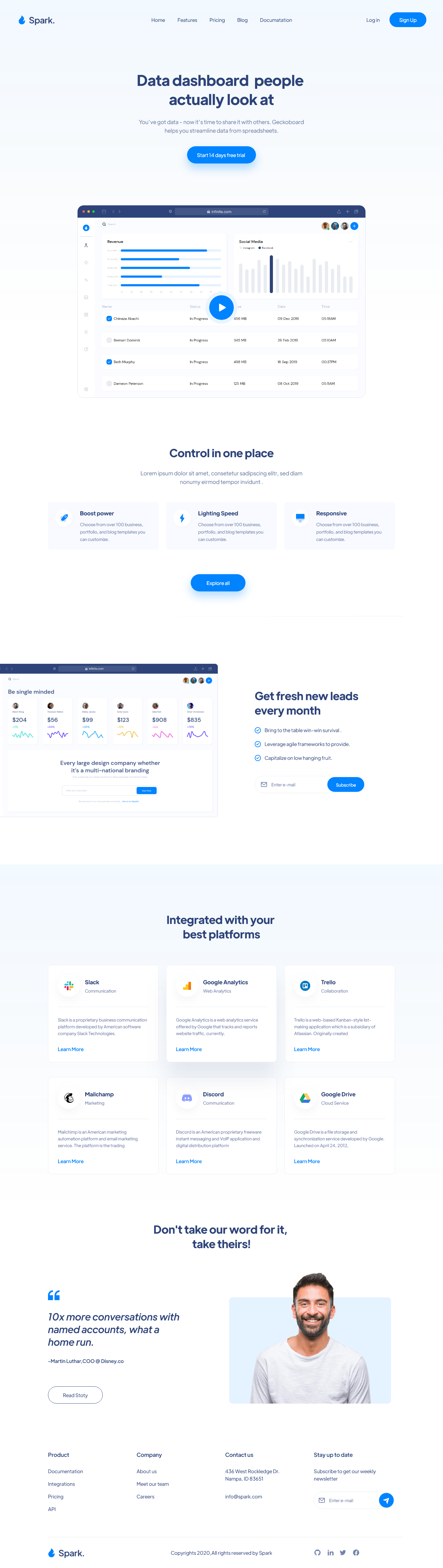This image is an extended screenshot from the website Spark, showcasing multiple views of its interface in a layered, collage-like arrangement. The website is designed with a light blue and white color scheme, giving it a clean and modern aesthetic. In the top-left corner, there is a box labeled "Spark," adjacent to another box featuring a blue tab that suggests a sign-up option.

At the top of the page, the menu prominently displays the phrase "Data Dashboard People Actually Look At," underscoring the website's focus on data visualization. Below this, there's a call-to-action menu offering a "Start 14 Days Free Trial" button, inviting users to experience the service firsthand.

The website emphasizes the importance of data sharing with a statement, "You've got data, now it's time to share it with others. GeckoBoard helps you streamline data from spreadsheets." This is followed by various examples of data visualizations, including different spreadsheets and widgets aimed at growing investments. 

Additionally, the screenshot highlights a section dedicated to customer reviews from other companies, praising Spark as the best website provider. Concluding the page, there's an extra quote at the bottom, further reinforcing the website's credibility and reliability.